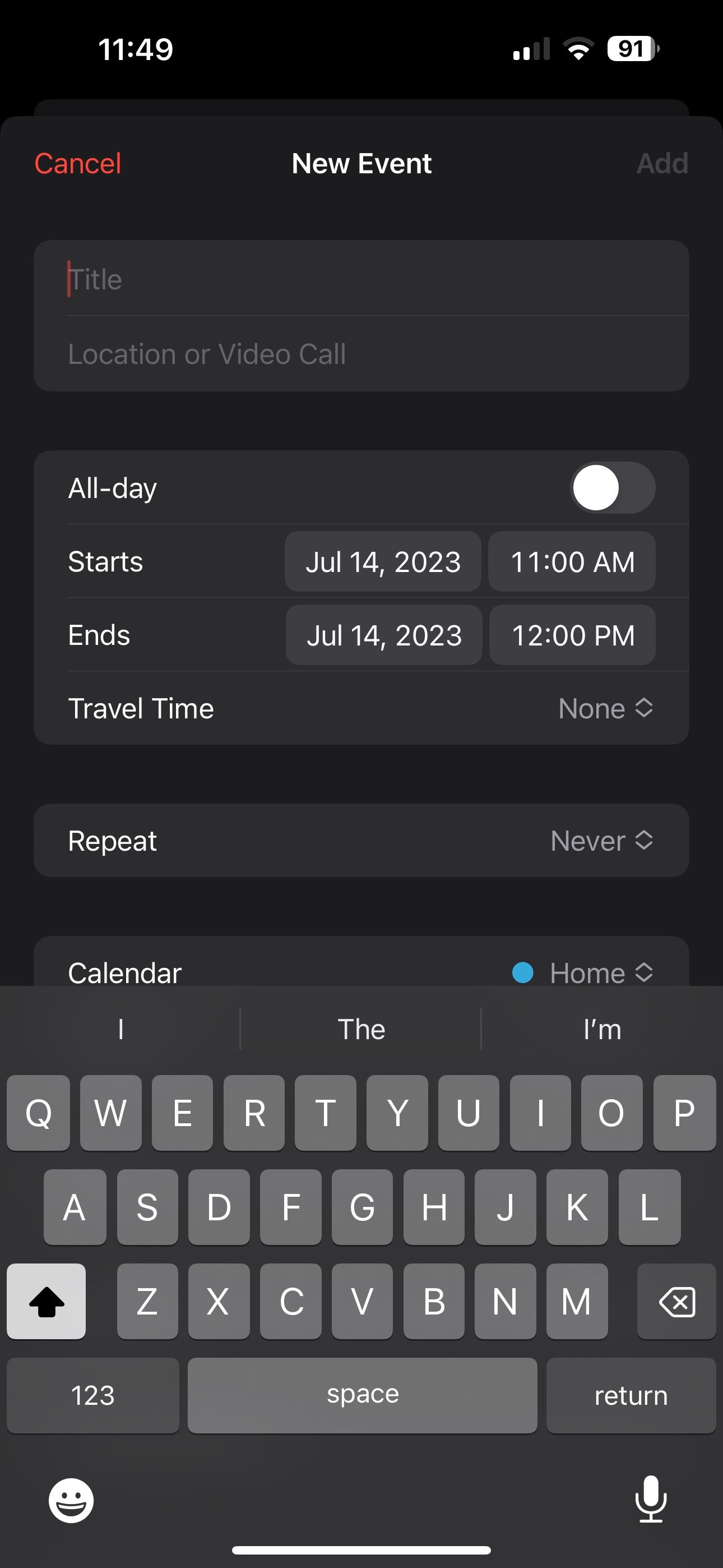The image is a detailed screenshot of a phone displaying a new event creation screen in a calendar application. The background is predominantly a dark charcoal gray, with several dark gray text fields and sections layered on top. At the very top, there is a black bar containing the options "Cancel" on the top left, "New Event" in the center, and "Add" on the top right corner.

Below this black bar, there are two primary text fields: the first labeled "Title" and the second labeled "Location or Video Call." Further down, several other fields are displayed:

1. "All-day" event toggle switch, currently set to off.
2. "Starts," which is set to July 14th, 2023, at 11 a.m.
3. "Ends," which is set to July 14th, 2023, at 12 p.m.
4. "Travel Time" with a dropdown menu, currently showing "None."
5. "Repeat" with a dropdown menu, set to "Never."
6. A calendar icon with a blue "Home" identifier.

The phone's keyboard is visible at the bottom of the screen, suggesting words across the top bar such as "I," "the," and "I'm." The keyboard itself has gray keys, encased in a light gray background with white lettering. At the bottom left of the keyboard, there's a smiley face emoji icon, while on the bottom right, there is a microphone emoji icon.